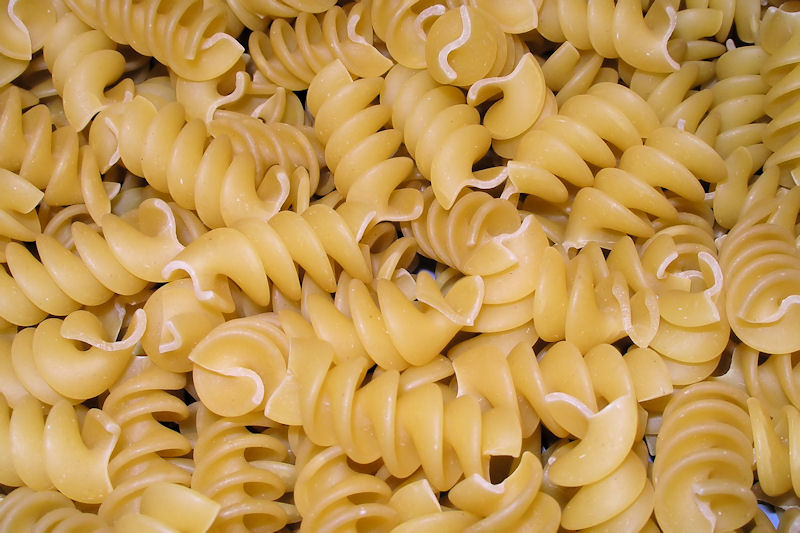This close-up photograph captures a heaped arrangement of spiraled pasta, showcasing approximately 30 to 50 light tan noodles. Each noodle displays five to six tight spirals, with their ends slightly lighter, suggesting where they have been cut. The focus is entirely on the intricate, twirled shapes of the pasta, highlighting the uniform texture and subtle color variations. The image is cropped closely to emphasize the detailed structure of the noodles, ensuring no other elements distract from the pasta's intricate design.